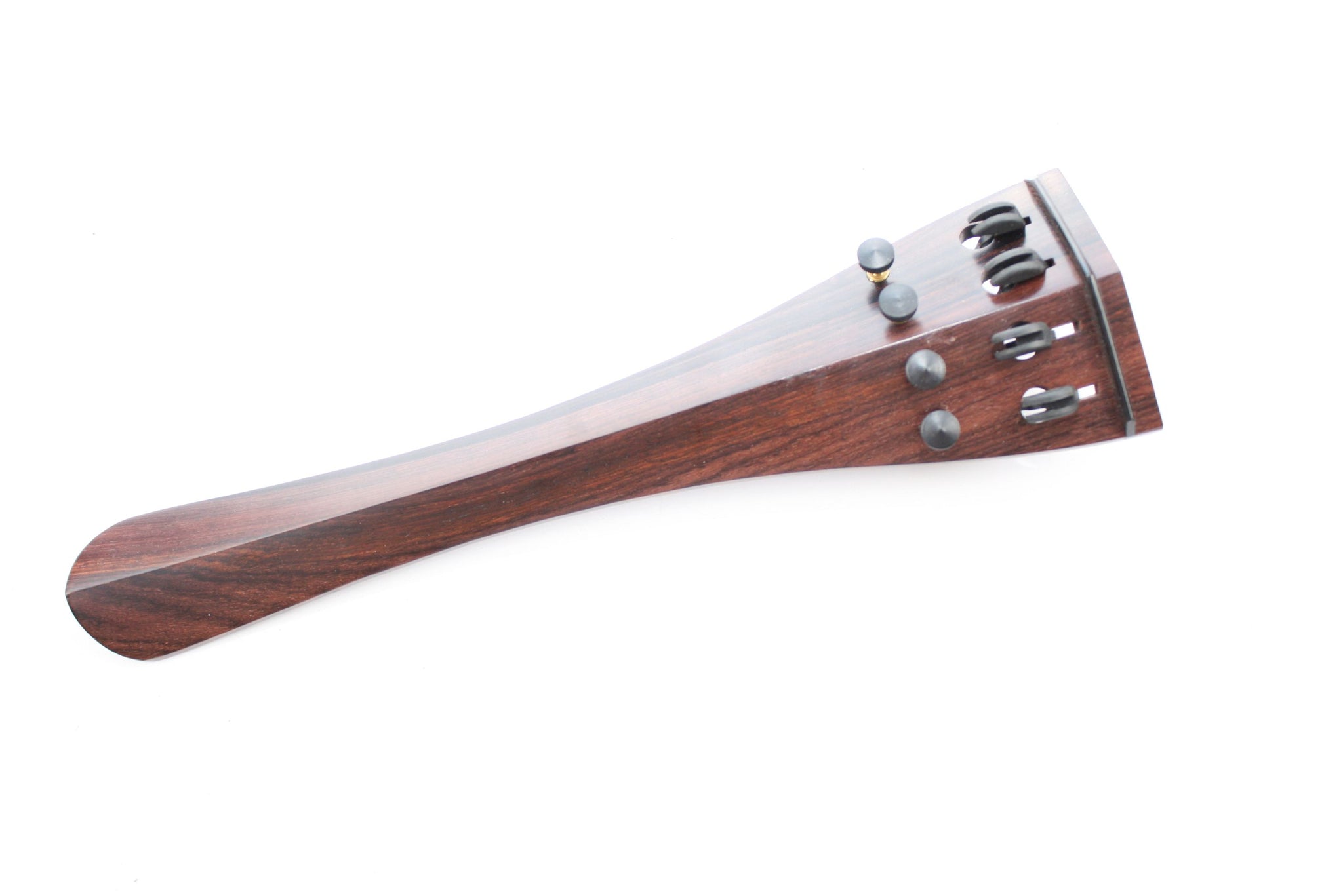The image showcases a finely crafted cello tailpiece made of smooth, light rosewood. This long and tapered wooden piece broadens at the base and features four tuning posts, which are used for delicate pitch adjustments. A distinct ridge runs along its middle, gracefully sloping downwards, and the top is accented with a piece of black metal that stretches across it. The tailpiece has four guides to hold the strings in place. Set against a white, featureless background that gives it a floating appearance, the high-quality photograph isolates the tailpiece entirely from the rest of the instrument, highlighting its detailed craftsmanship and design.